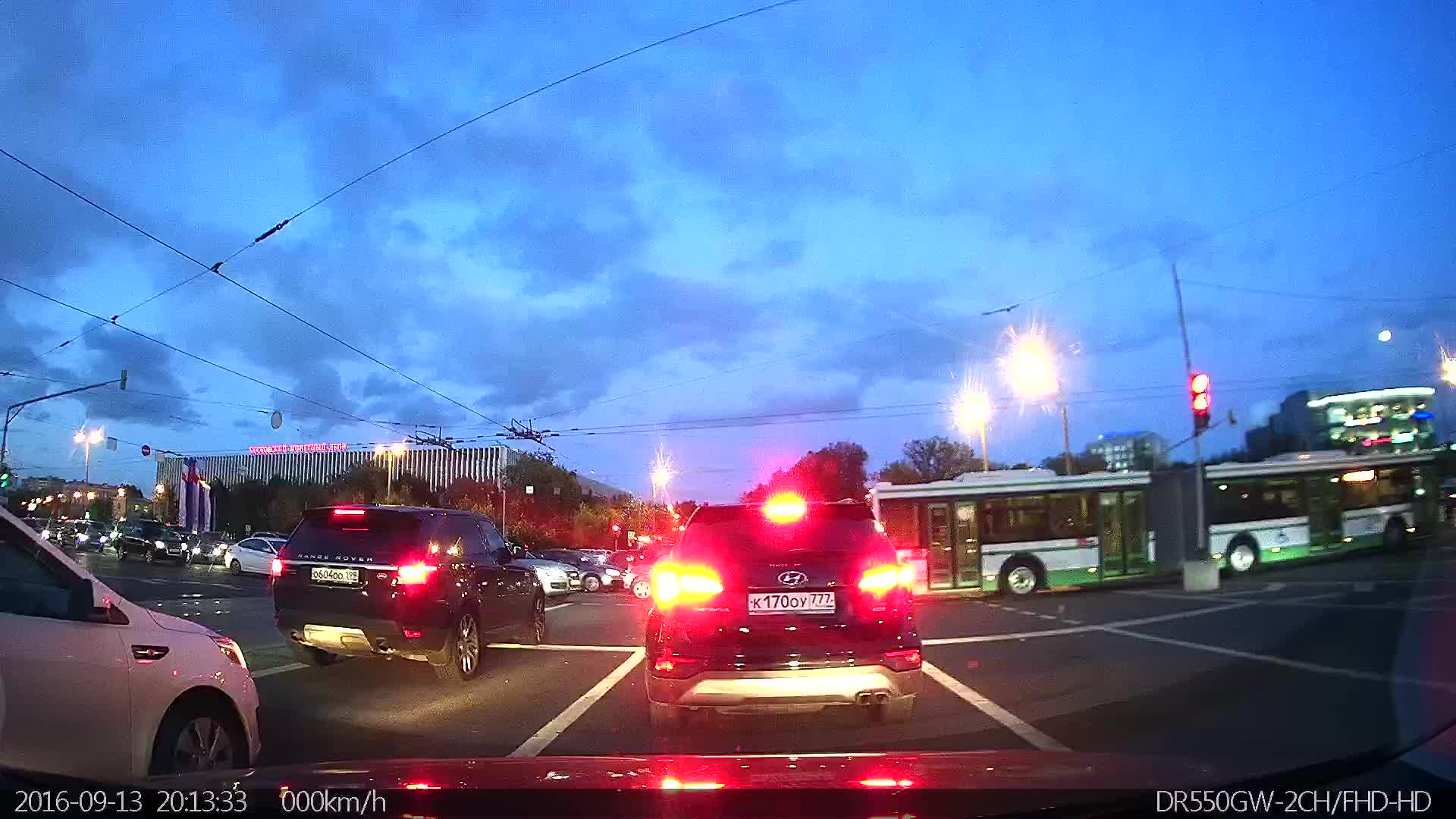This horizontal, rectangular photograph captures a bustling suburban intersection at dusk, where traffic is at a standstill. The sky is a vibrant blue with dark clouds, signifying the end of the day. In the foreground, you can see the top of the photographer's car. Two SUVs are directly ahead, their bright brake lights creating a glare. A smaller white car is positioned at the lower left corner. 

The road is filled with numerous vehicles, including a long white and green double bus, which can be seen driving from the right side towards the left. The road surface is dark with visible white stripes, suggesting a formal street layout rather than a parking lot. Utility wires stretch overhead, and various streetlights and building lights illuminate the surroundings. 

On the left side, a large, tall building is noticeable, though the writing on its roof is illegible. The intersection itself is broad, with multiple lanes filled with cars coming from and heading in various directions, implying heavy traffic flow. 

Printed in white text on the bottom left corner of the image are the details "2016-09-13," "20:13:33," and "0 KM/H," indicating that the photograph might have been taken from a police car's dashcam. In the bottom right corner, there is a longer string of identifying text: "DR-550GW/2CHFHDHD."